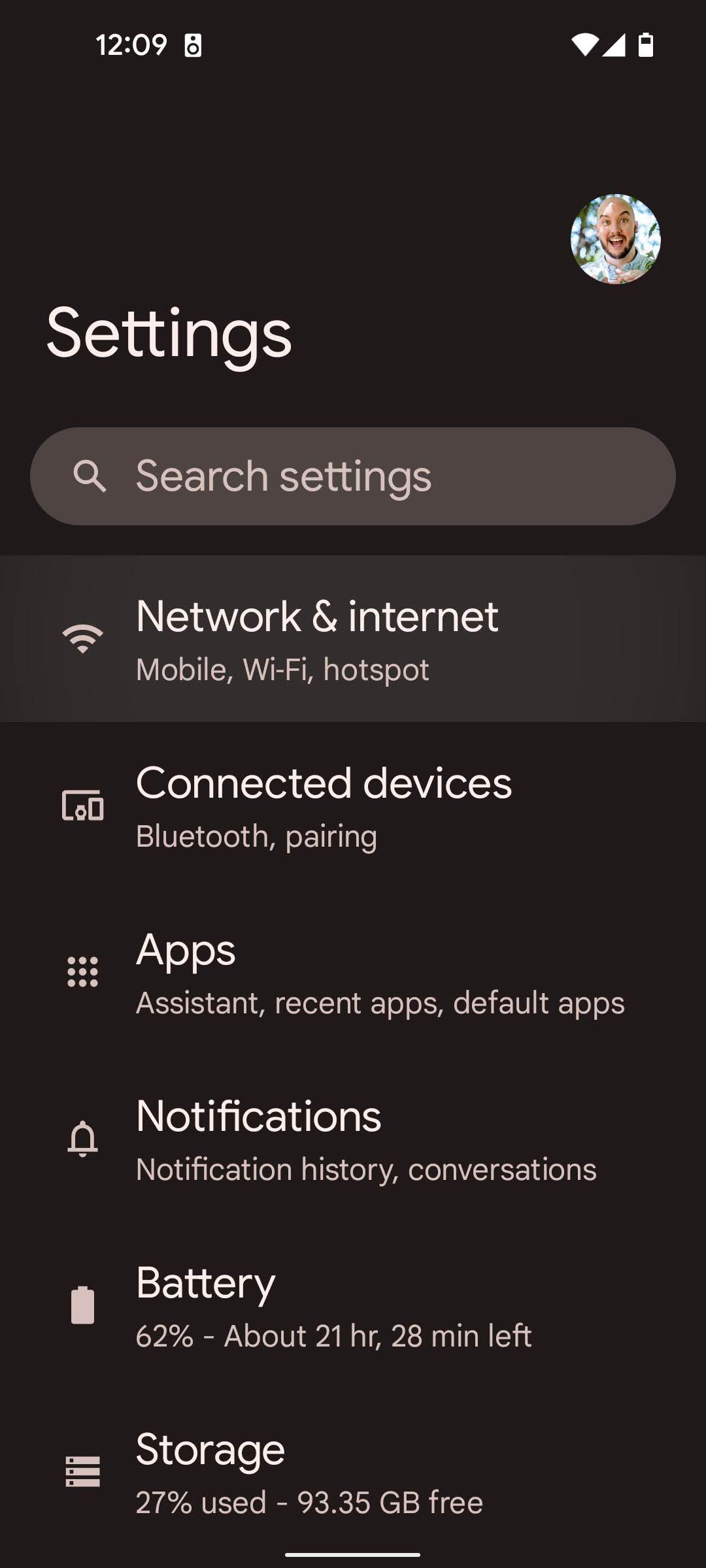The image is a screenshot taken from a mobile device, with a solid black background and white text. In the top left corner, the time is displayed as 12:09, while the top right corner shows Wi-Fi status and a battery level at three-quarters full. Below these indicators, within a circular frame, is a photo of a young man with a bald head, dark brown beard, and mustache. He is smiling broadly and wearing a bright, flowered shirt.

To the left of the circular image is the word "Settings." Below this, there is a search box labeled "Search settings."

In a vertical list, the following categories and their subcategories are detailed:
- Network & Internet: mobile, Wi-Fi, hotspot
- Connected devices: Bluetooth pairing
- Apps: Assistant, recent apps, default apps
- Notifications: notification history, conversations
- Battery: 62%, about 21 hours and 28 minutes left
- Storage: 27% used, 93.35 gigabytes free

The entire layout is concise, visually neat, and designed for easy navigation and quick access to various settings and information.